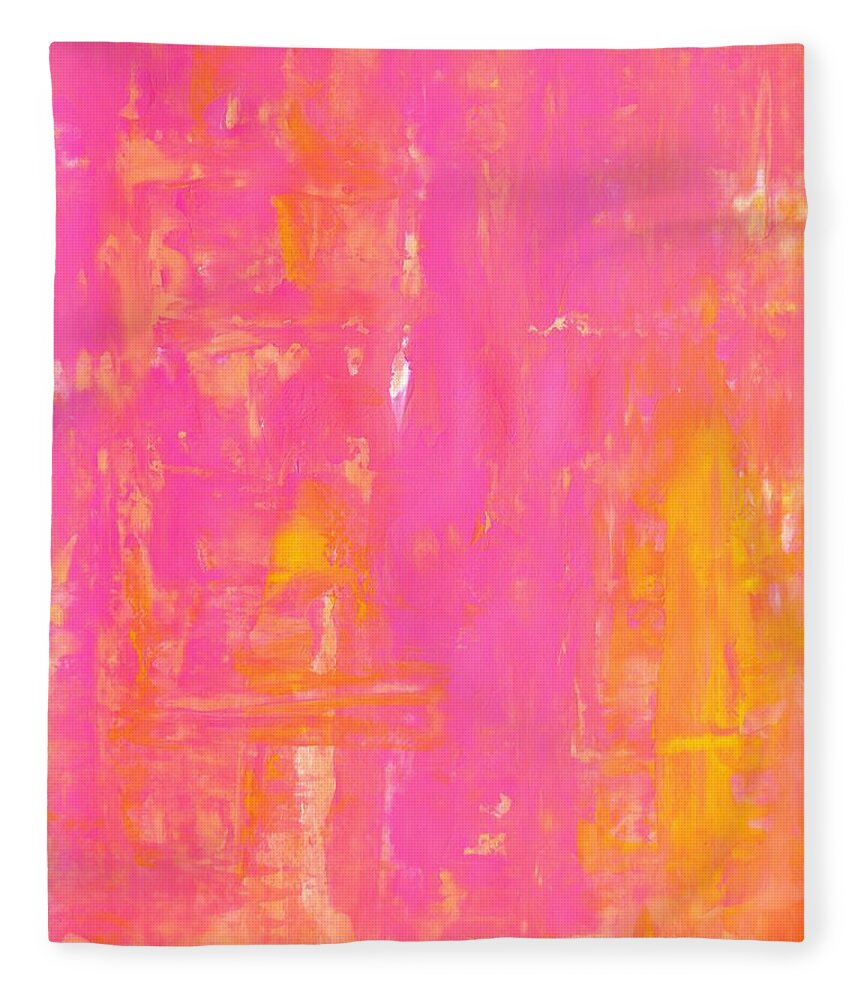The image depicts an abstract watercolor painting that evokes a dreamlike or nightmarish atmosphere. Dominated by a swirling mix of pink, yellow, and orange hues, the painting features layers of color that blend and smear together in vertical and horizontal strokes. While primarily using pink for the background, the bottom right corner showcases vibrant splashes of yellow and lime green, and the lower left corner transitions into shades of pink and orange. Though the painting lacks any distinct objects or text, some viewers have noted the presence of abstract forms that could be interpreted as a pair of eyes in the upper right section. Despite the absence of a visible signature, the image exhibits the kind of intricate and imaginative design often found in museum pieces by artists with elaborate visions.